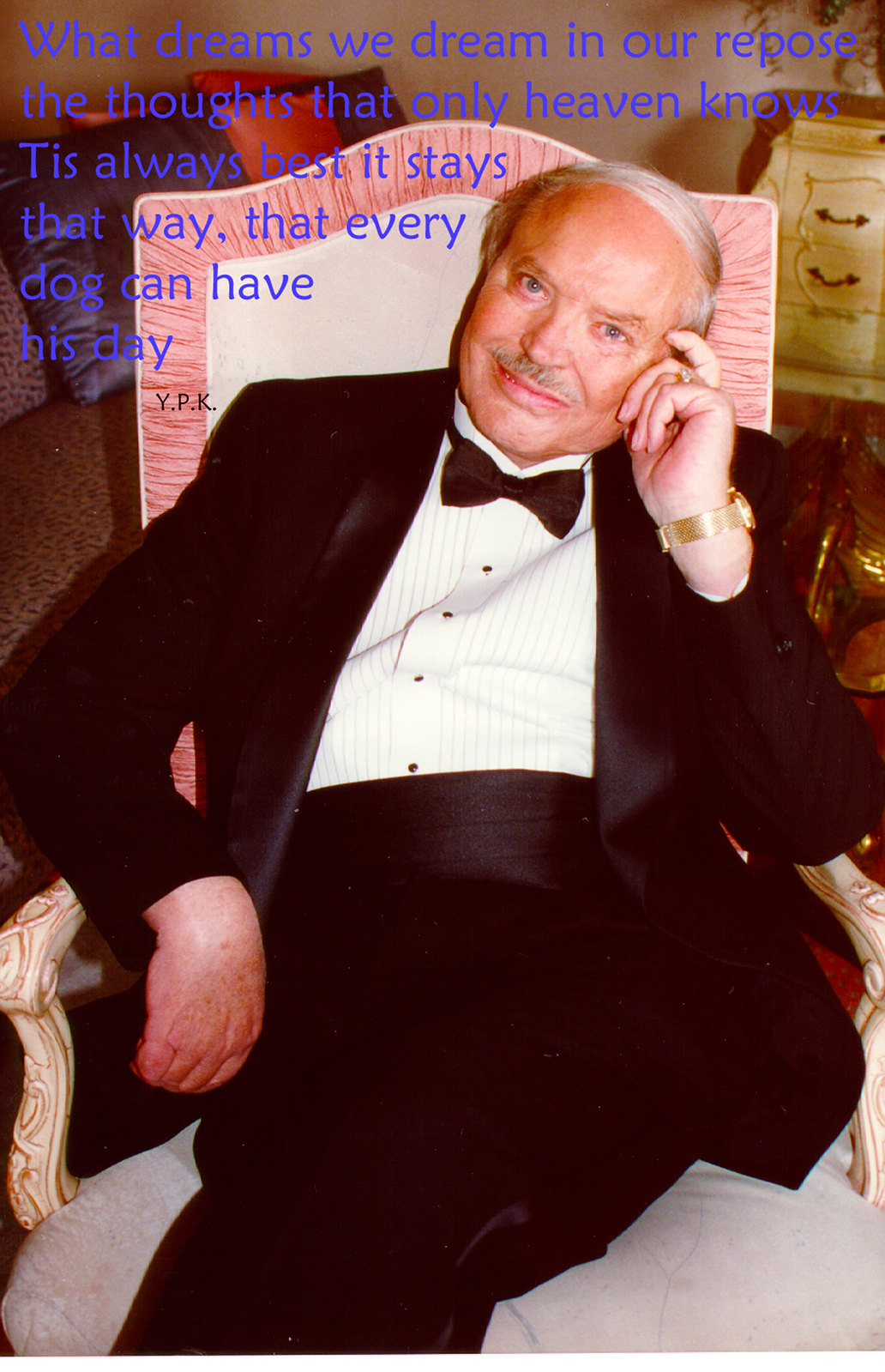The image features an older man dressed in a sophisticated black tuxedo, complete with a white shirt and black bow tie, complemented by a golden watch on his wrist. He sits in an ornate chair with a high back, adorned with a white cushion and a light brown frame, accented by a pink, frilly edge. The man, slightly smiling, poses with his finger pointed at his temple while resting his head on his left hand. In the background, there is a small dresser and blurred colors that hint at furniture and a wooden floor. Superimposed in blue text at the top of the image is the quote: "What dreams we dream in our repose, the thoughts that only heaven knows. It is always best it stays that way, that every dog can have his day." Below this, at the bottom right, the initials "YPK" are written in black text. The overall scene exudes an air of elegance and contemplation.